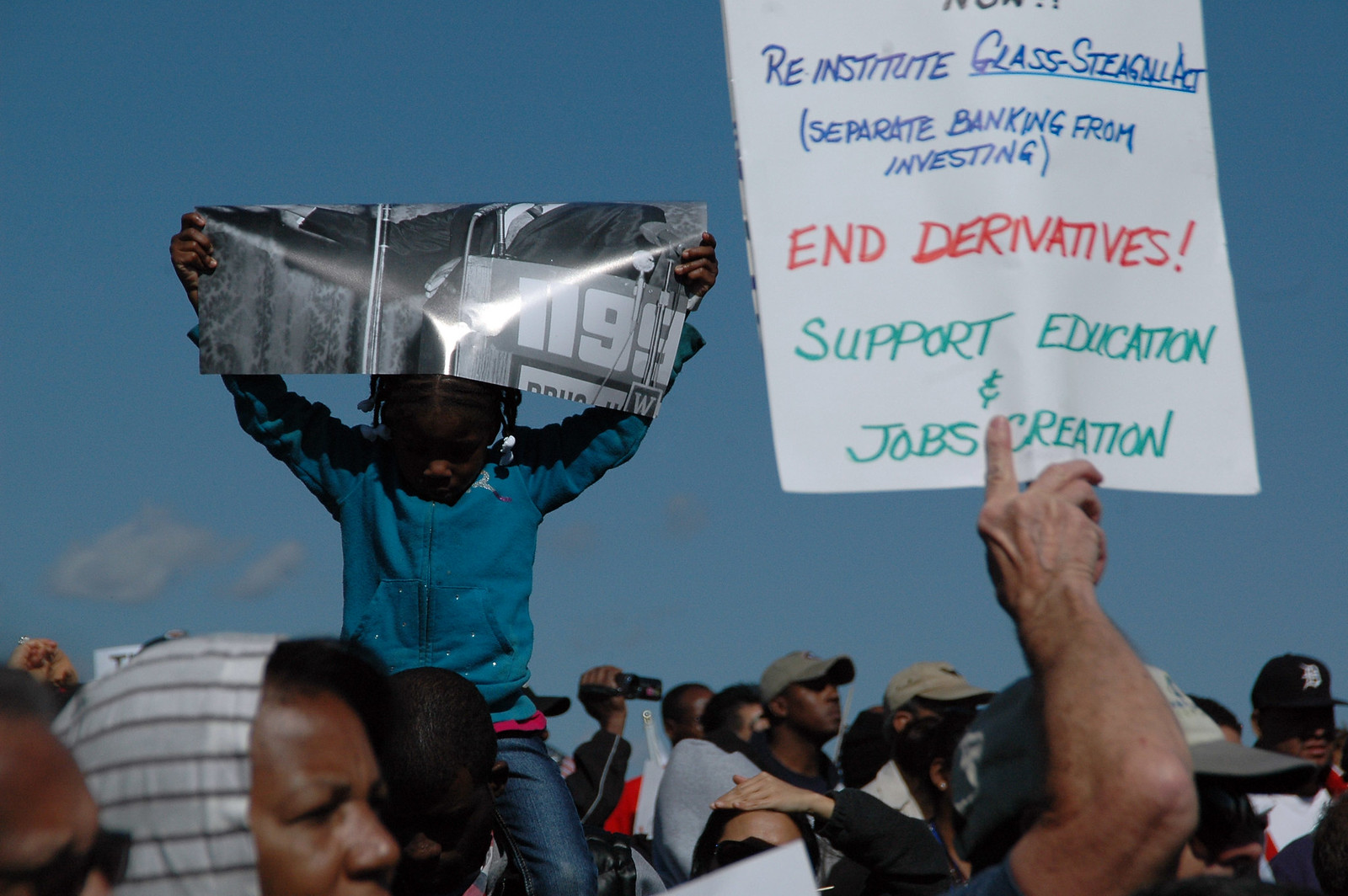The image depicts a large outdoor public demonstration, seemingly a protest or strike. Central to the scene is a young boy wearing a blue hoodie, perched on a man’s shoulders. He is prominently holding up a black-and-white photo of someone in a suit, partially obscured, with the inscription "N99" visible below it. To the right of the boy, an adult holds a vertical white sign adorned with messages written in blue, red, and green marker. The top portion is cut off, but the visible text reads: "reinstate Glass-Steagall Act," followed by "separate banking from investing," "end derivatives," and "support education and job creation." Many people in the crowd are looking in various directions, contributing to the dynamic atmosphere of the protest.